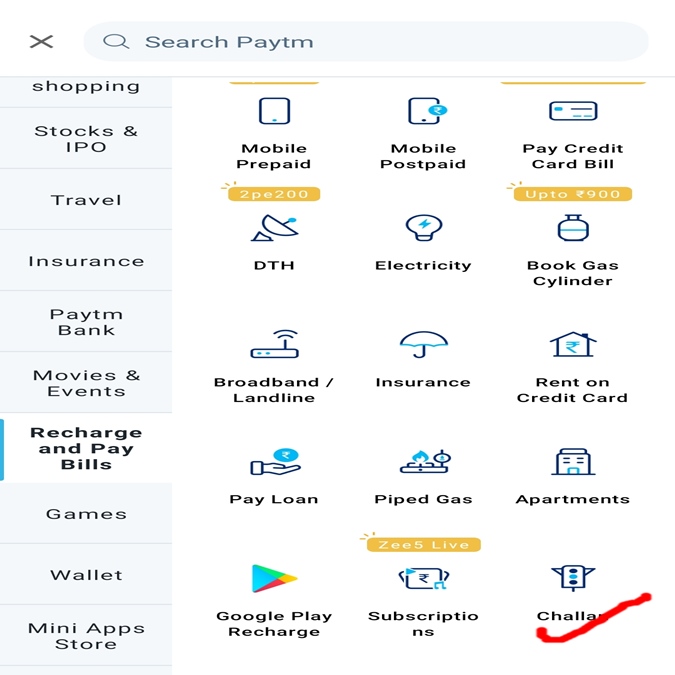In this image, there's a detailed view of a digital interface, presumably from the Paytm app. The interface features a side menu positioned on the left side, characterized by a light grey background and black text. The side menu includes various options like "Shopping," "Stocks and IPO," "Travel," "Insurance," "Paytm," "Bank," "Movies and Events," "Recharge and Pay Bills," "Games," "Wallet," "Mini App Store," among others. The "Recharge and Pay Bills" option is currently highlighted in white with a blue line accentuating its left side.

The top section of the interface includes a search bar labeled "Search Paytm." The main content area on the right is divided into various sections.

- At the top, there are categories such as:
  - **Mobile Prepaid**, highlighted by the text "2 PE 200" and an orange buzzer.
  - **Mobile Postpaid**.
  - **Pay Credit Card Bill**, with a note mentioning "up to 900 rupees" and marked in brown.

- Subsequent sections include different services:
  - **DTH** on the left.
  - **Electricity** in the center.
  - **Book gas cylinder** on the right.
  - **Broadband Landline** on the left.
  - **Insurance** in the center.
  - **Rent on Credit Card** on the right.
  - **Pay Loan**.
  - **Piped Gas**.
  - **Apartment** on the right.

At the bottom left of the interface, there is a Google Play recharge option, represented by a triangular Google Play icon in blue, green, red, and orange, facing to the left. Additionally, there are options for "Subscription," "Challenge," and "Challah," the latter featuring a red outline with a matching red checkmark.